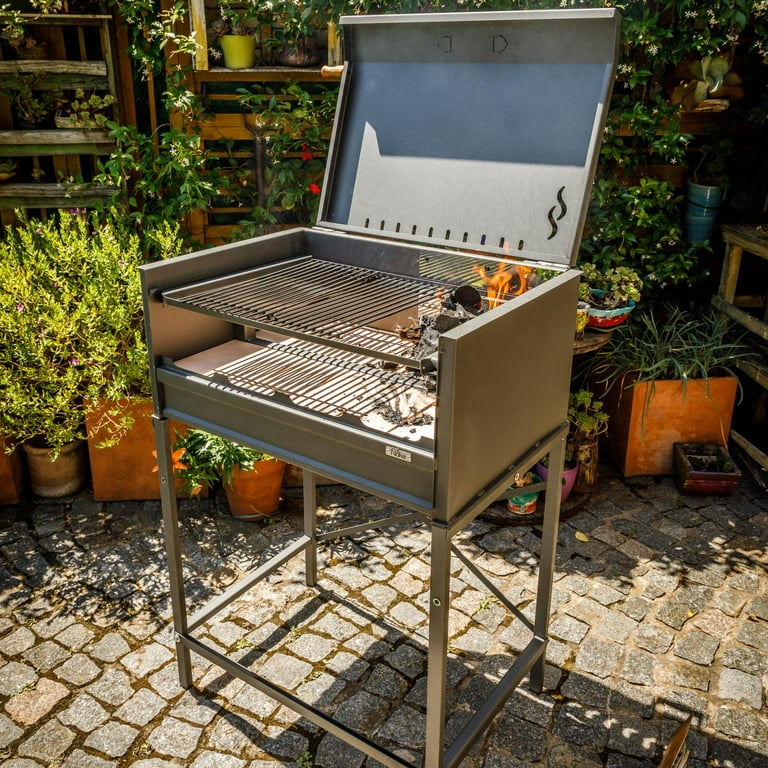The image depicts a sunny outdoor scene in a backyard or garden with a gray, two-tiered barbecue grill situated on brick cobblestone pavers. Flames are visible on the right side of the grill, and although the specific items on the grill are unclear, a logo featuring two squiggly "S" shapes, possibly representing flames, is present on the lower right-hand corner of the lid. Surrounding the grill are a plethora of potted plants, including various small-leafed and spiky varieties, arranged on shelves and the ground. Some plants behind the grill even display blooms. Ivy is also visible around the overall structure. In the background, there are wooden elements, such as a railing or ladder, further enhancing the garden ambiance.